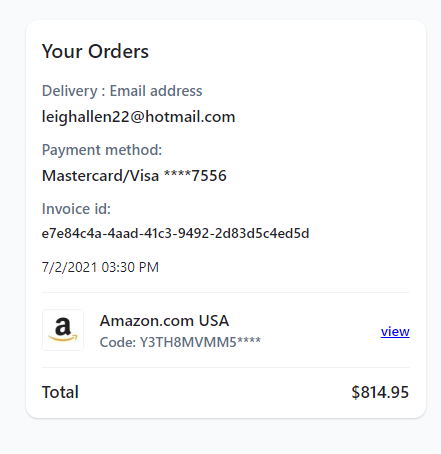In the photograph, we observe a detailed screenshot of an order confirmation from Amazon. Dominated by a white background and black text, the top of the image prominently displays "Your Orders" in bold black lettering. Below this header, in gray text, are the words "Delivery, Email Address," followed by the black text of the email "LeighAllen22@hotmail.com."

The payment method for this order is indicated as "MasterCard Visa," with the card details partially obscured by asterisks, revealing only the last four digits: 7556. An invoice ID is presented, consisting of a series of alphanumeric characters separated by spaces, though the specific characters are not clearly visible in the description.

This order was placed on July 2, 2021, at 3:30 PM. The recognizable Amazon logo—a stylized "A" in black with a yellow arrow underneath—is also present, reaffirming the source as "Amazon.com USA." A notable blue hyperlink labeled "View" is visible, presumably allowing the user to access more details about the order.